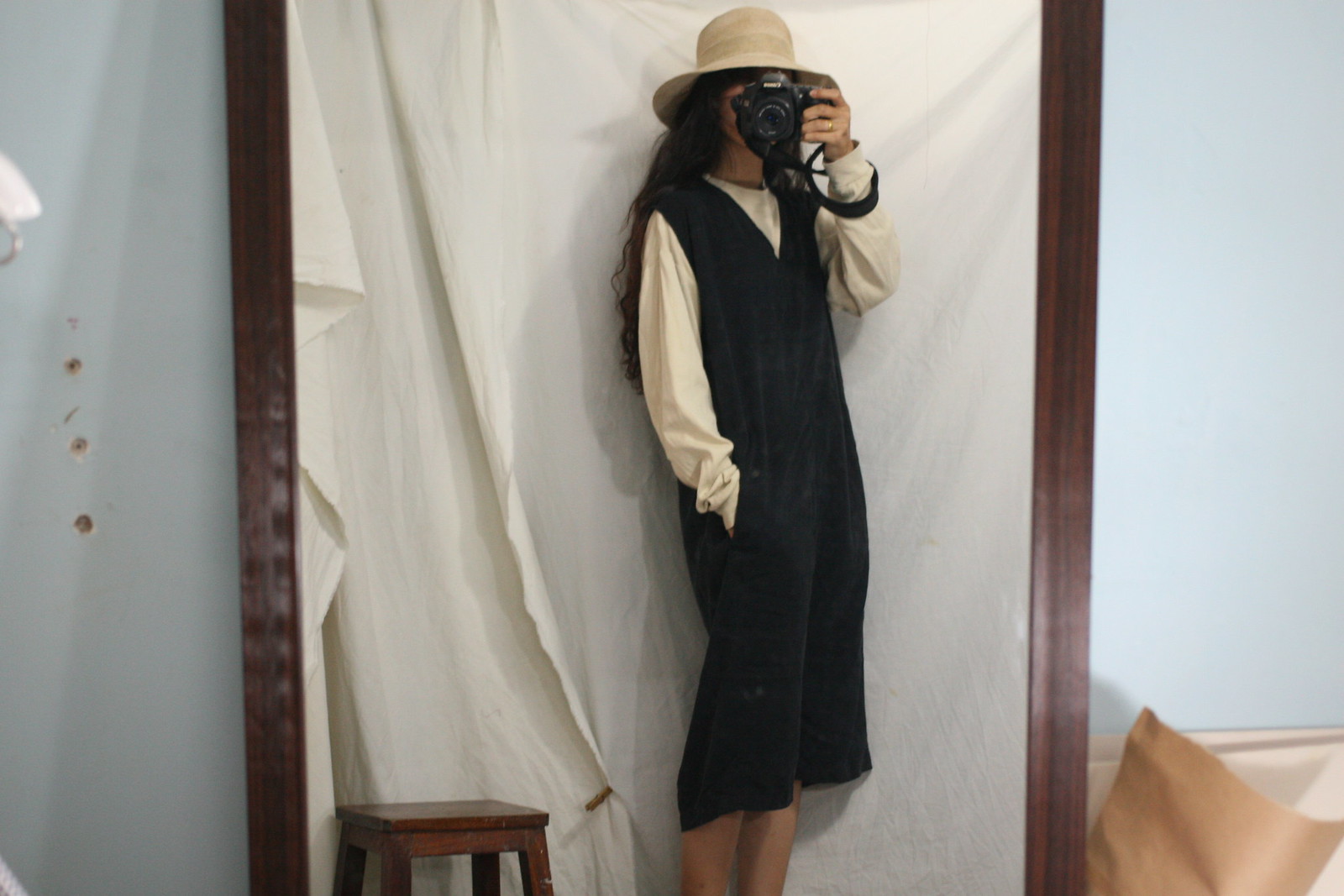This image captures a woman taking a self-portrait using a large DSLR camera in front of a wide mahogany-framed mirror. The camera, held in her left hand, obscures her face, but you can see her long, dark brown hair cascading beneath a beige sun hat. She's dressed in a black dress layered over a baggy, flowy white long-sleeve shirt. In the reflection, behind her, there is a white sheet that appears to be fastened with a clothespin, and part of the background includes a light blue painted wall with some imperfections, such as small holes. Additionally, there is a small brown stool visible in the bottom left corner, and part of a couch or chair with an orangish pillow on it. The clear and simple brown-framed mirror highlights her and the aesthetic details of the room.